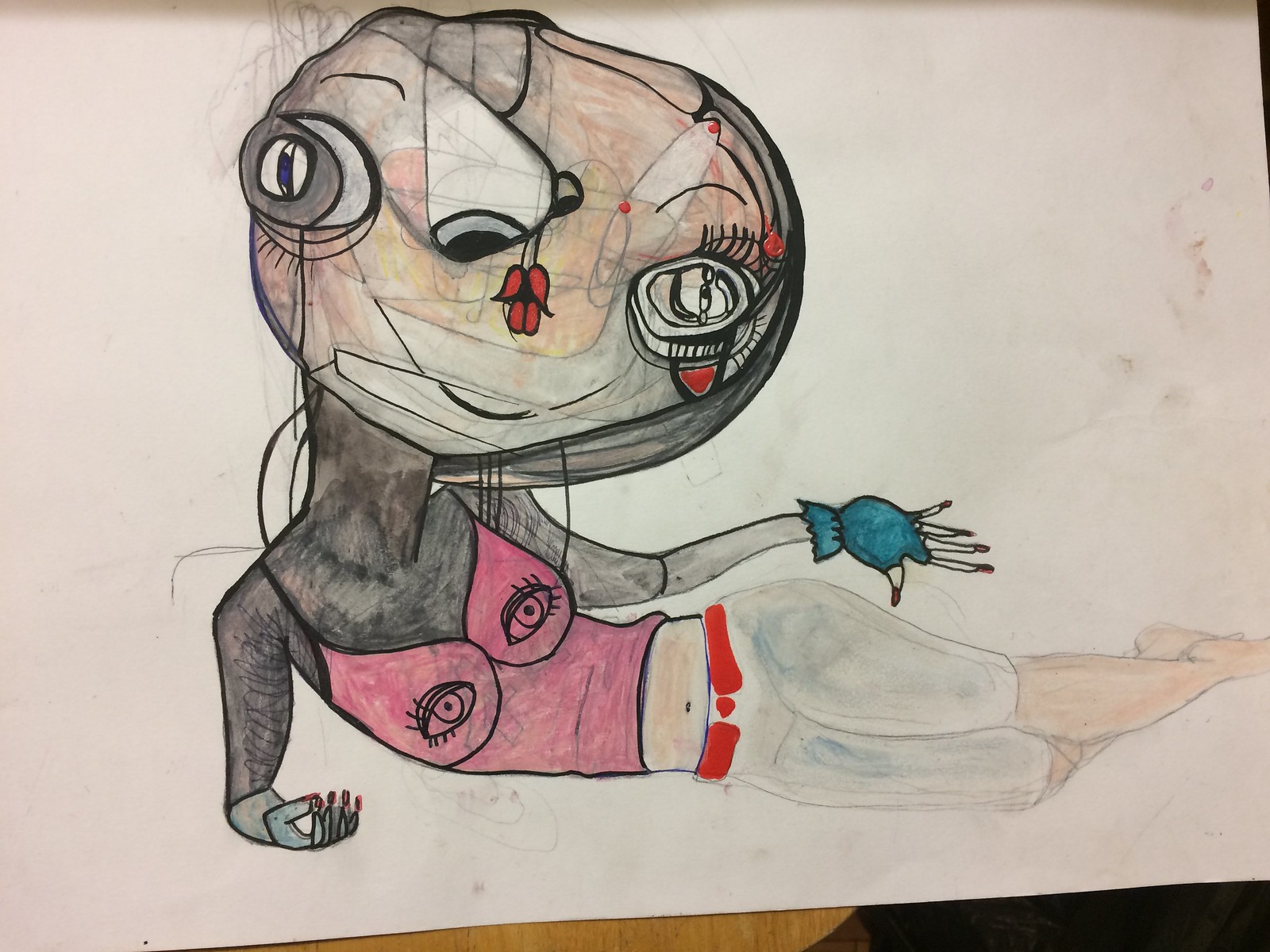This image captures a photograph of a drawing sketched on white paper. The artwork depicts a creatively stylized humanoid figure with distinct and varied features. The figure’s head is oval-shaped, featuring two asymmetrical eyes: one is thin, blue, and slit-like, while the other has numerous lashes and is colored gray. The facial features, including the nose and mouth, appear deliberately distorted. 

The humanoid’s body is portrayed with a grayish skin tone. It is dressed in a pink shirt adorned with eye motifs on the upper part. The shirt leaves the midriff exposed, and the lower half of the figure is illustrated wearing white pants with a red belt. The figure is positioned on its side, creating a relaxed and unconventional pose. A green glove adorns its left hand, adding an additional splash of color to the ensemble. The overall composition highlights a blend of vibrant colors and abstract elements, reflecting a unique artistic vision.